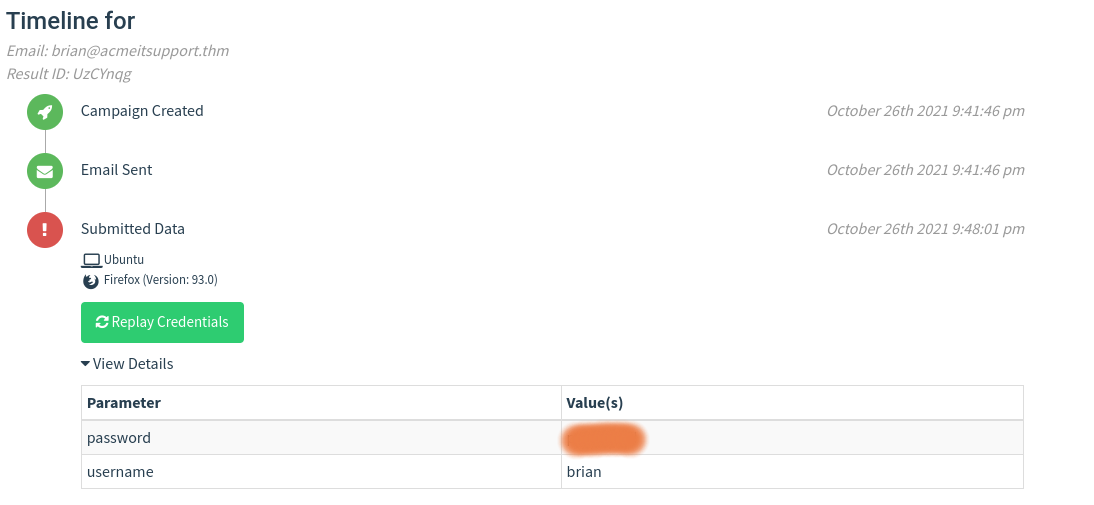The image illustrates a detailed timeline of an event sequence. Against a white background, the title "Timeline 4" is prominently displayed. It also includes an email address, "brian@acmetsupport.thm," and an identifier label, "Result ID: UZC Young." 

The timeline starts with a green circle containing an airplane icon labeled "Campaign Created." A line extends downward to another green circle featuring an envelope icon with the label "Email Sent." Further down, a smaller line connects to a red circle with an exclamation point icon, marked "Submitted Data."

Adjacent to this sequence is a small computer screen displaying the details: "UB, Unread 2, Firefox version 33.0." Below, a green button labeled "Replay Credentials" and another button "View Details" with a downward arrow are present. 

The image also includes two boxes: one labeled "Parameter" with fields for "Password" and "Username," and another labeled "Values." There is a brown oblong box containing the name "Brian."

On the right side, at the top, there are three timestamps: "October 26, 2021, 9:41:46 PM," "October 26, 2021, 9:41:46 PM," and "October 26, 2021, 9:48:01 PM."